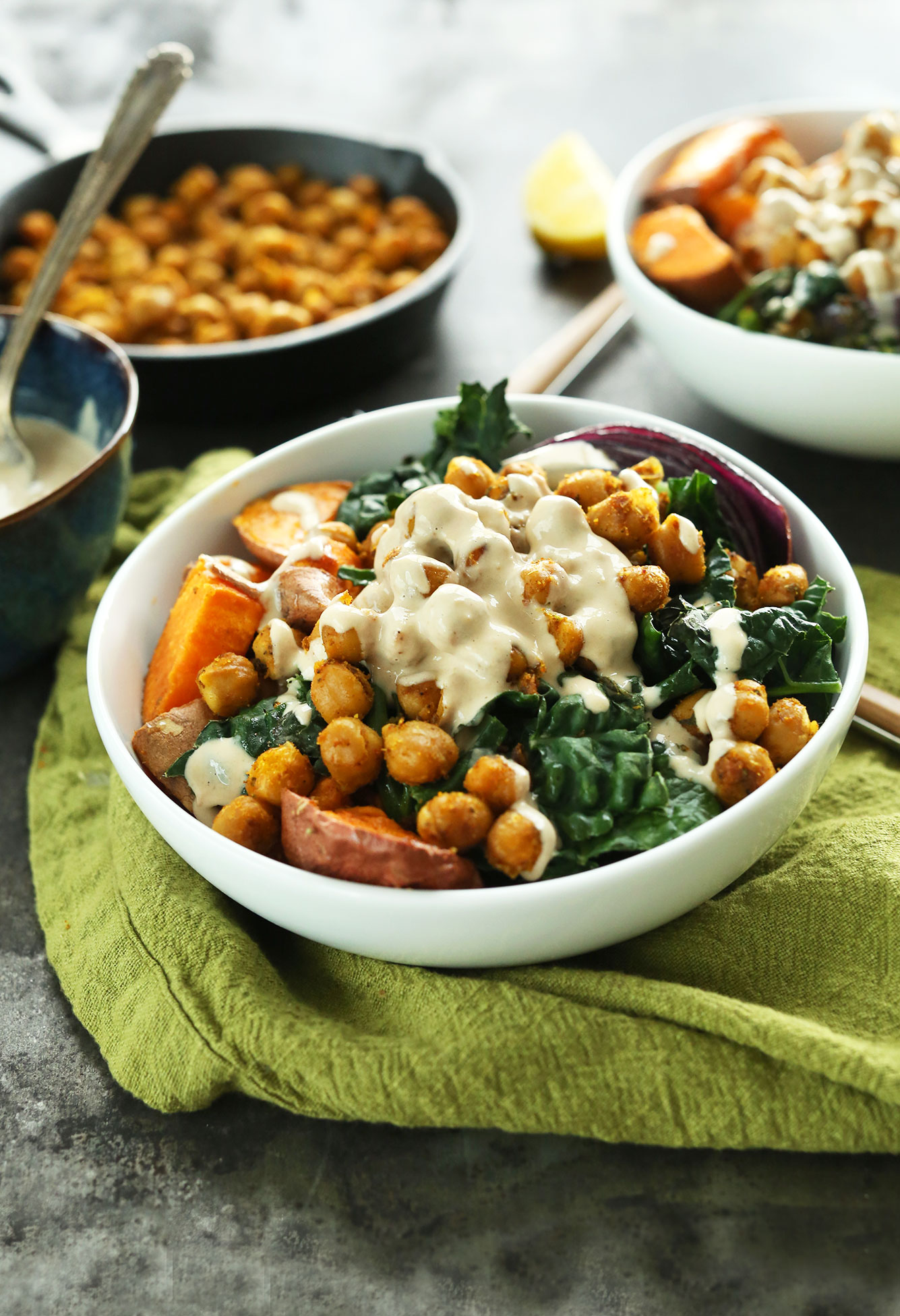In this detailed image, a vibrant bowl of salad takes center stage, placed on a green towel atop a gray marble countertop. The main salad, housed in a pristine white ceramic bowl, features a hearty mix of chickpeas, dark leafy greens—likely spinach or kale—and chopped sweet potatoes. The ensemble is generously drizzled with a creamy white salad dressing. A hint of red onion and possibly some croutons add texture and complexity to the dish. Surrounding the feature bowl are three additional bowls. To the left, a smaller bowl holds what appears to be salad dressing, complete with a spoon resting in it. In the background, partially blurred, a white bowl contains a similar salad mixture, positioned beside a segment of sliced lemon. Behind these, a black bowl or skillet is filled with chickpeas, suggesting they were pre-cooked. Finally, another dark bowl, also blurred, showcases a salad sans cheese but otherwise similar in composition to the main bowl. The array of colors—green, white, yellow, and dark hues—along with the elements of the picture, creates a visually appealing scene of a well-prepared, wholesome meal.